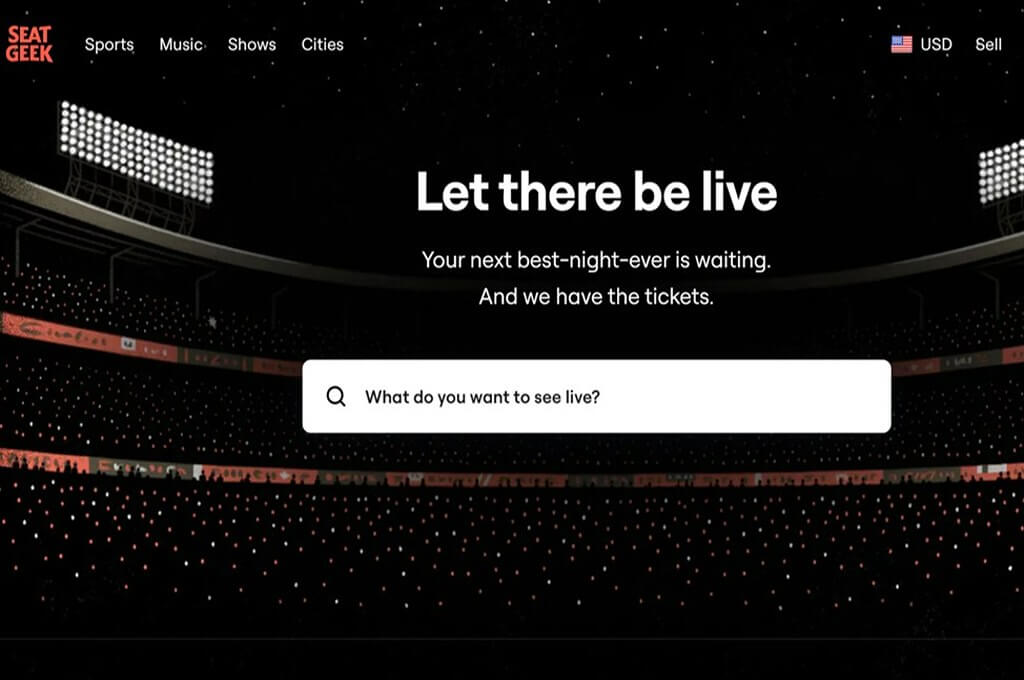The image depicts a vibrant nighttime scene set against a black background, resembling a soccer stadium. At the top, the brand "SeatGeek" is prominently displayed in bold red lettering. Below this, a white menu bar lists categories including "Sports," "Music," "Shows," and "Cities." An American flag icon accompanies the text "USD" and "SALE." 

A prominent slogan in the image reads, "Let There Be Love," followed by the tagline, "Your next best night ever is waiting, and we have the tickets." This emphasizes the company's promise to provide memorable experiences. 

At the center, a search bar with a magnifying glass icon to its left invites users to query, "What do you want to see live?" 

The background features a black sky filled with an array of twinkling stars, adding to the atmospheric charm. The scene is further illuminated by two bright stadium lights, enhancing the liveliness of the depicted venue.